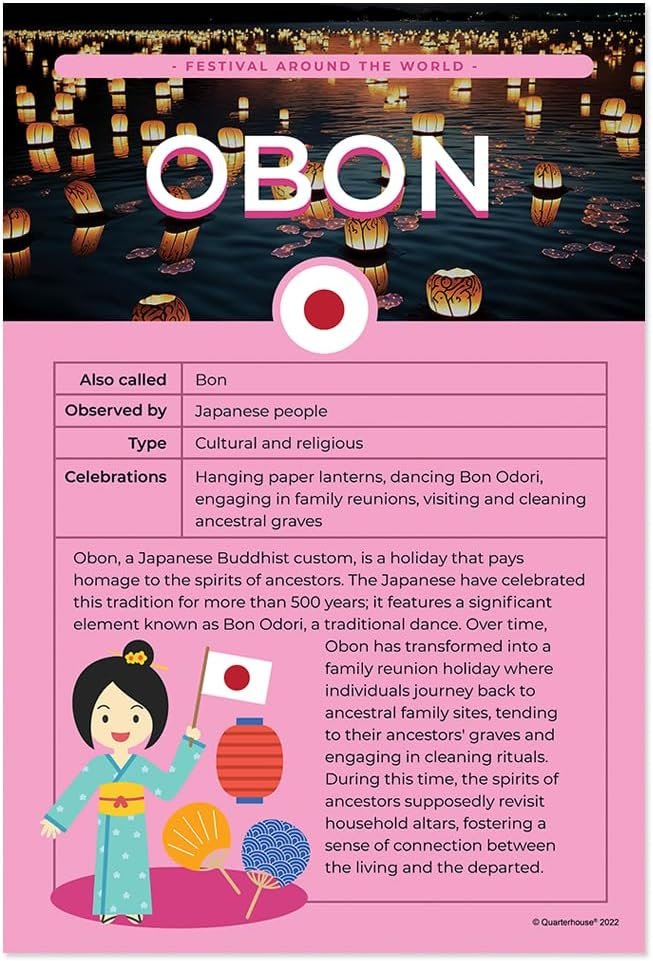This vibrant and informative poster explains the Japanese festival of Obon, also called Bon. Set against a purple background, it features a photo at the top depicting paper lanterns floating in water among lily pads, with bold text in white and pink that reads "OBON" and a pink banner declaring "Festival Around the World." The text explains that Obon is a Japanese Buddhist custom observed by Japanese people and is both a cultural and religious event. Celebrations include hanging paper lanterns, dancing the traditional Bon Odori, and participating in family reunions and cleaning ancestral graves. Obon has been celebrated for over 500 years, serving as a holiday to honor the spirits of ancestors. The traditions associated with Obon foster a deep sense of community and connection between the living and the departed. Additional details note that the festival features table blocks or informational sections that describe its significance. In the bottom left corner, there is a clip art-style cartoon illustration of an Asian woman in a kimono, holding a Japanese flag, accompanied by a paper lantern and two fans. The bottom right corner of the poster includes the small text "Quarter House 2022."